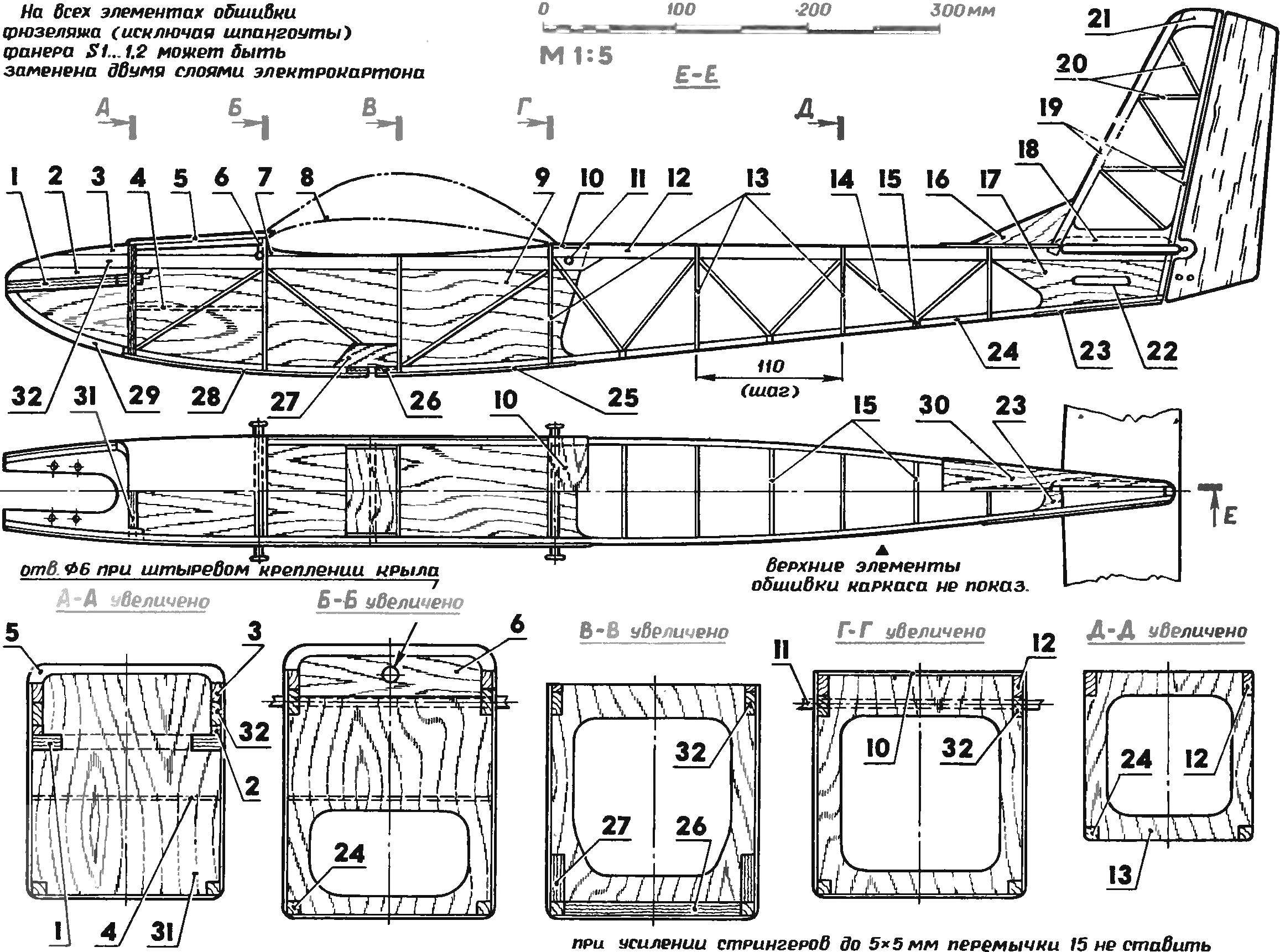The image depicts a detailed black-and-white blueprint of a wooden airplane model, highlighting its various components. The blueprint prominently features a scale at the top center, ranging from 0 to 300 millimeters, with a note indicating that the scale is 1:5. Surrounding the airplane frame, which lacks an engine and features a clear canopy at the front, are around 32 to 33 parts, each meticulously numbered and labeled. In the top left corner, Cyrillic text spans four lines, providing additional context, though the specifics remain untranslated. Below the scale and scattered across the diagram are multiple smaller illustrations, possibly close-up views or section breakdowns, each accompanied by further numbering and labeling to aid in the assembly process. The blueprint serves as an intricate guide for constructing this wooden aircraft model, detailing every element from the fuselage to the tail with precision.